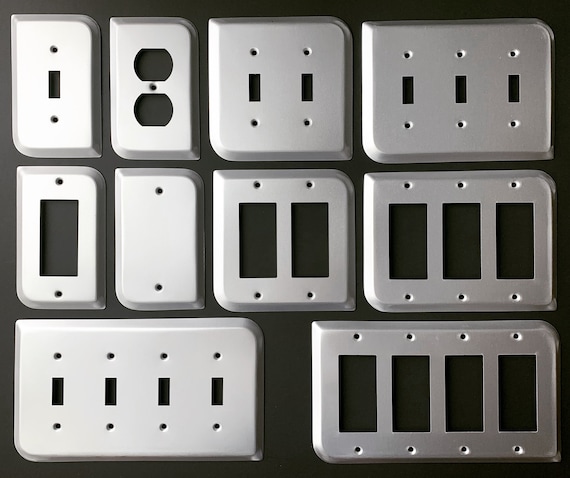This image is a highly detailed, color photograph taken from an overhead perspective, capturing an assortment of roughly ten light switch and socket outlet plates in various shapes and sizes. The plates, fabricated from chrome or stainless steel, exhibit a consistent design with curved top left corners and rounded edges. They are meticulously arranged in three rows on a black background, typical of product photography with a focus on realism.

In the top row, a single switch plate is positioned next to a double plug-in switch plate, both following the same corner design. Moving to the center row, a rocker switch plate is placed on the left, flanked by a blank plate, with double and triple switch plates adjacent to it, all maintaining uniform corner configuration and stainless steel finish.

The bottom row features two four-plate switch covers, differentiated by the types of switch openings: smaller standard switch openings on the left and rocker switch openings on the right. The standout details include the precise holes in each plate for screws, indicating where they are to be affixed to the wall. These elements, devoid of any text or words, underscore the utilitarian yet meticulously detailed nature of the photograph.